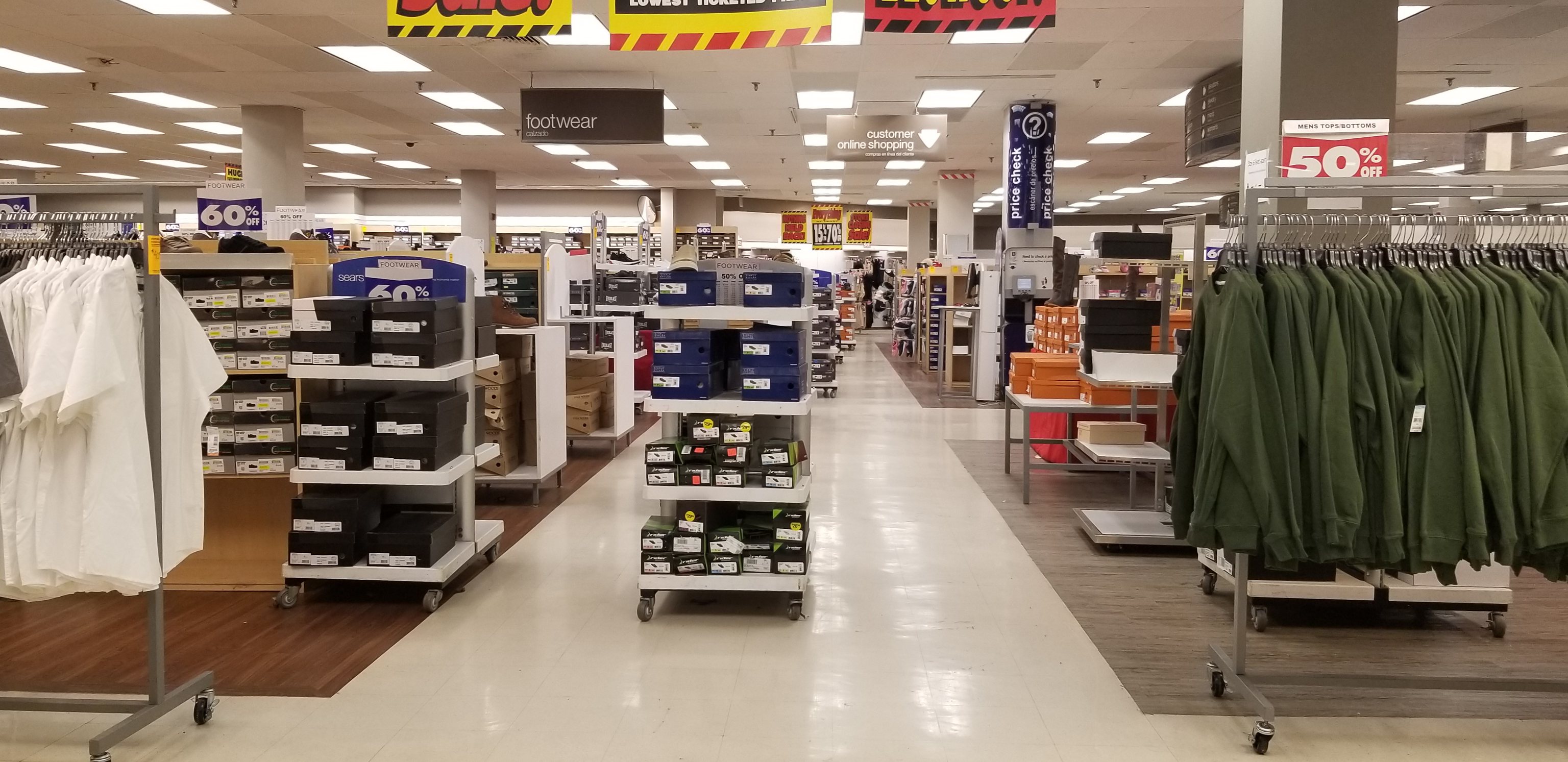The image showcases a meticulously organized retail store. Prominently featured are three upper signs, though only their bottoms are visible. The first sign is yellow with red and black text, the second also yellow with red and black text, and the third, predominantly red with black writing. On the right side of the store, a "50% off" sign is visible above racks adorned with green-colored clothing. Contrastingly, on the left side, there are racks displaying short-sleeve white shirts. As you move further inside, there is a footwear section marked with a "60% off" sign. In the background, matching signs to those at the front are present, though their text is unreadable from this vantage point. The store's floor is predominantly white, but the sections have distinct flooring: brown on the left and gray on the right. The overall appearance is exceptionally tidy and well-maintained.